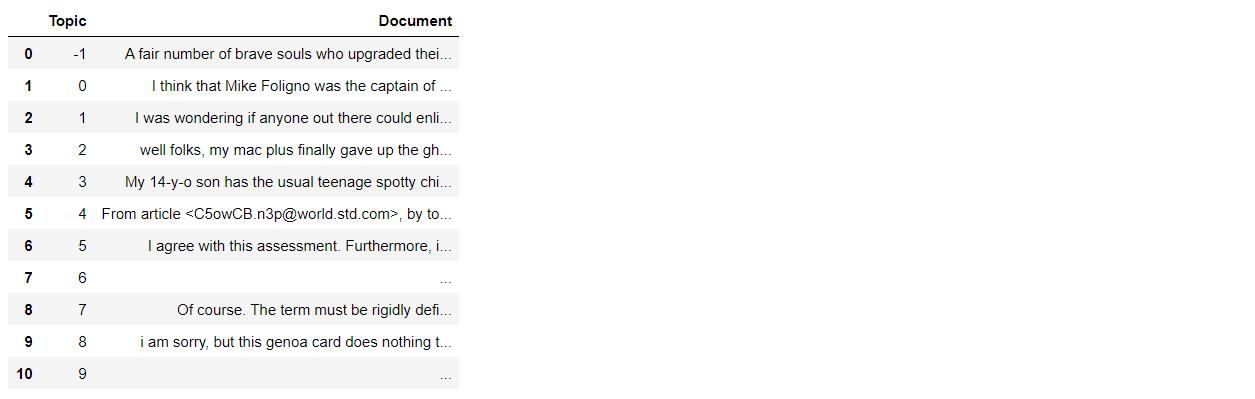The image depicts a webpage that is noticeably off-center, skewed to the far left of the frame. The webpage lacks a clear title or description, diving straight into its content. At the top, there are headers labeled "Topic" and "Document." Below these headers, the content consists of a numbered list, each entry beginning with a numerical identifier followed by fragmented text. The list includes:

1. A sentence about brave individuals who upgraded their devices, possibly with reference to someone named Mike Falagina as captain.
2. A question posed, seeking assistance or listing something.
3. A statement about a Mac Plus computer that has ceased functioning.
4. A comment involving a 14-year-old teenager with typical spots.
5. An article that provides a specific number.
6. An agreement with an unspecified assessment.
7. A blank entry.
8. A declaration about items needing to conform strictly.
9. A complaint about a general card that is ineffective.
10. Another blank entry.

The numbers are followed by text that is cut off and incomplete. The webpage is presented in a monochrome color scheme, with alternating white and gray shaded bars for each entry, giving a segmented yet unclear visual structure. The overall context and purpose of the webpage remain ambiguous due to the truncated text.